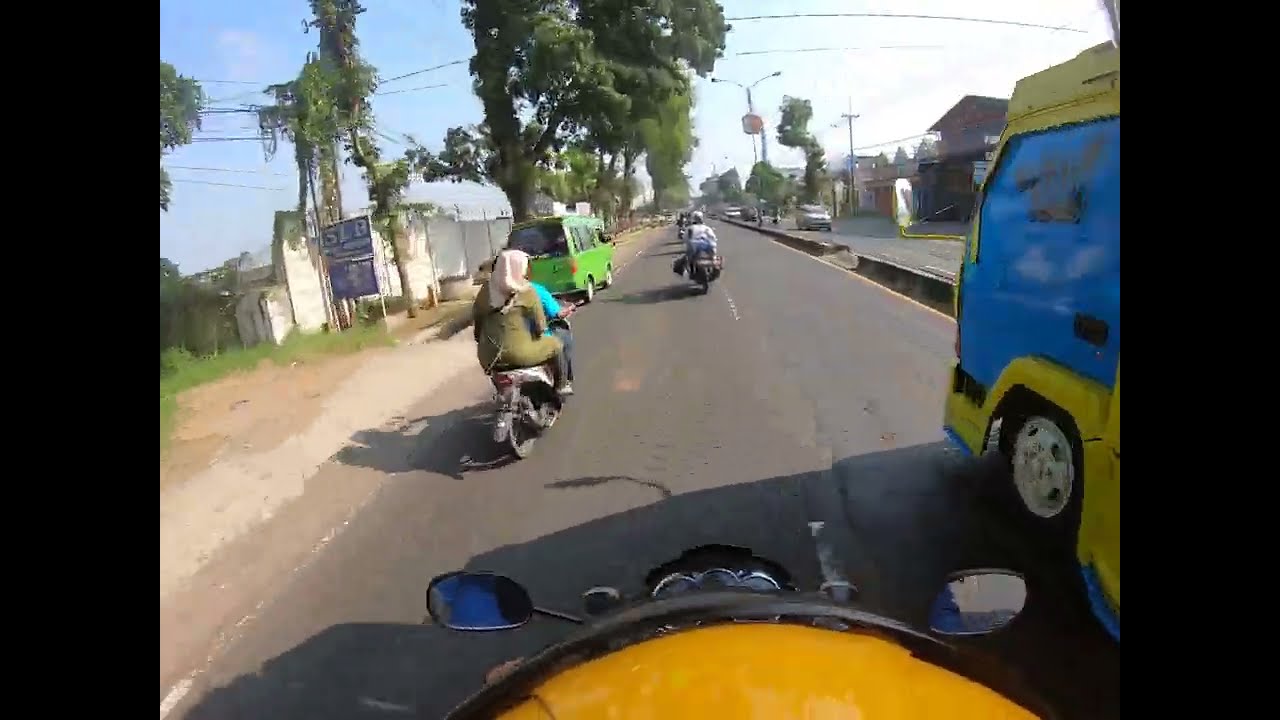The photograph, taken from a GoPro mounted on a motorcycle, captures a bustling street scene, presumably in a European country given the left-hand traffic. The camera angle is slightly tilted to the left, revealing a dynamic view of the surroundings. Two mirrors at the lower part of the image feature yellow ovals indicating the motorcycle's presence. 

Ahead, a couple of scooters are riding in the left lane, one of which carries a woman with a beige kerchief. The green minivan is parked along the left side near a small shack. The busy street contains several vehicles: a blue bus or van is visible on the right, and numerous street cars are parked along the roadside. Trees and small homes line the street, contributing to a scenic yet urban atmosphere. To the right, another lane of traffic flows in the opposite direction, under a clear blue sky subtly transitioning to a hazy ambiance on the right.